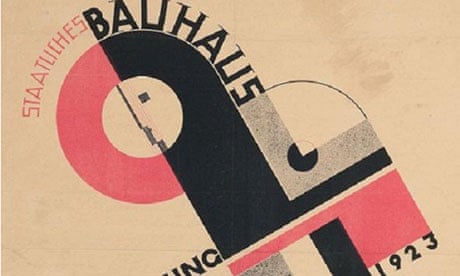This is an illustration from 1923, possibly advertising or referencing the Bauhaus movement, featuring a blend of geometric shapes and text. The background is a creamish, taupe color, slightly yellowed with age, evoking a vintage feel. 

At the top left, the words "Staatliches" in pink and "Bauhaus" in black are prominently displayed in capital letters. Below this, a circle is divided with the left half in pink and the right half in black, extending downward in a shape that integrates rectangles and arcs. Notably, a gray and white square intersects the top center of the circle.

The illustration includes elements suggesting an abstract, creature-like form constructed from geometric figures. The composition appears tilted slightly to the left, enhancing its dynamic appearance. The year "1923" is situated at the bottom right in black, while partially visible letters, "ING," are at the bottom left, hinting at a cutoff word. The colors used primarily include dark gray, light gray, black, and pink, adding depth and contrast to the design.